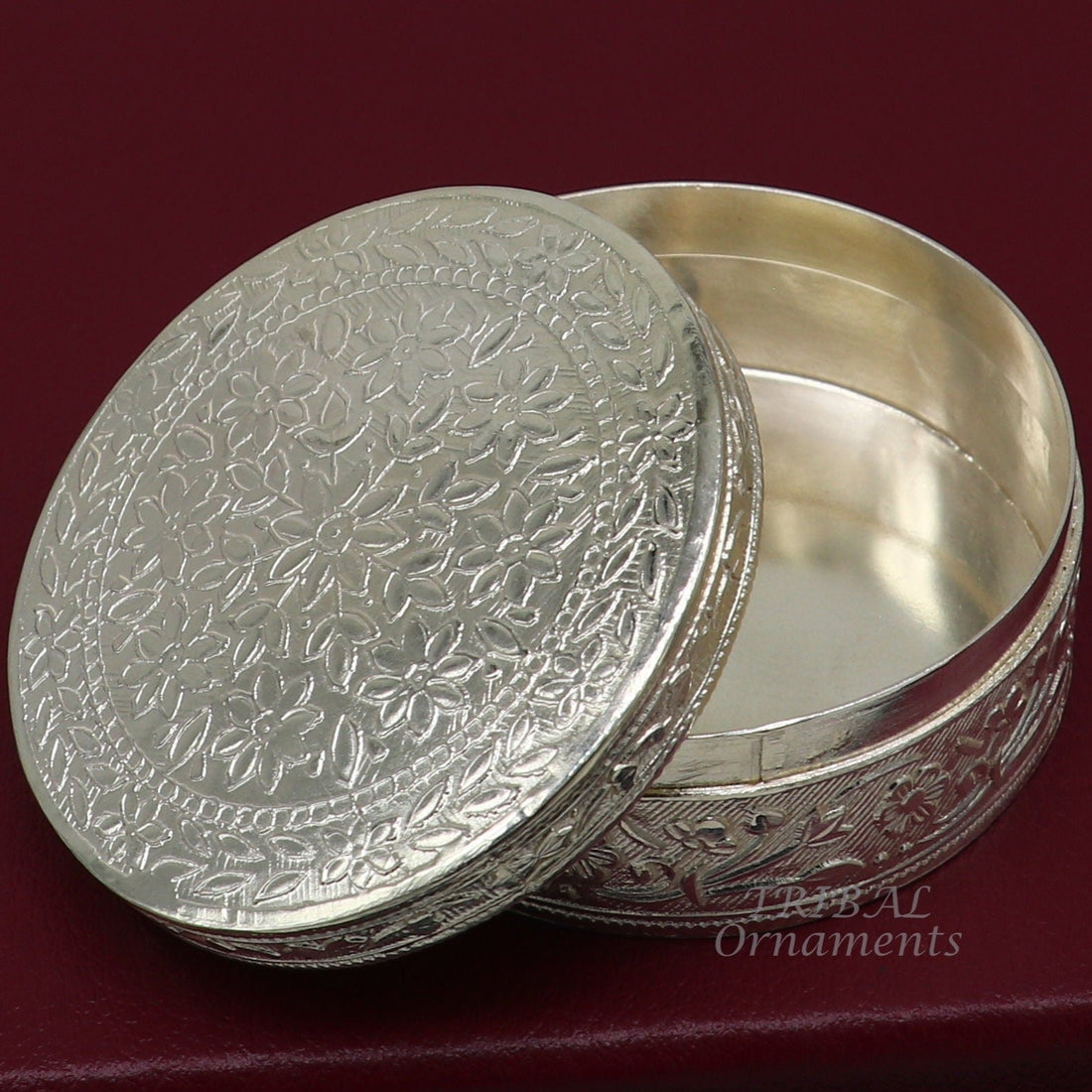The realistic photograph features a highly ornamented, vintage-looking silver round tin resting on a smooth, deep cherry-colored wooden surface. The tin, reminiscent of an old snuff or tobacco container, measures approximately six to eight inches in diameter and about two to three inches high. Both the lid and the cylindrical base of the tin are adorned with intricate engravings of flowers, leaves, and decorative wheat stalks, giving it an ornate and antique appearance. The lid is partially off, revealing a smooth interior. In the bottom center right of the image, there is a faint watermark reading "tribal ornaments."